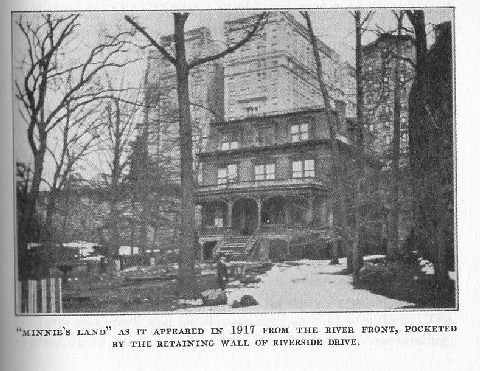This grainy black-and-white photograph, likely taken during the daytime, dates back to 1917 and is captioned "Minnie's Land as it appears in 1917 from the riverfront, pocketed by the retaining wall of Riverside Drive." At its center lies an image of a three-story home with a wooden porch supported by pillars, accessible via a staircase. The home also features two upper levels adorned with windows. In the vicinity of the house, barren trees and a walkway are visible, with a lightly snow-dusted yard and multiple trees on either side. Behind the house, three large, probably apartment buildings loom, adding to the urban landscape. A barely discernible person stands outside the house, seemingly clad in a black suit.